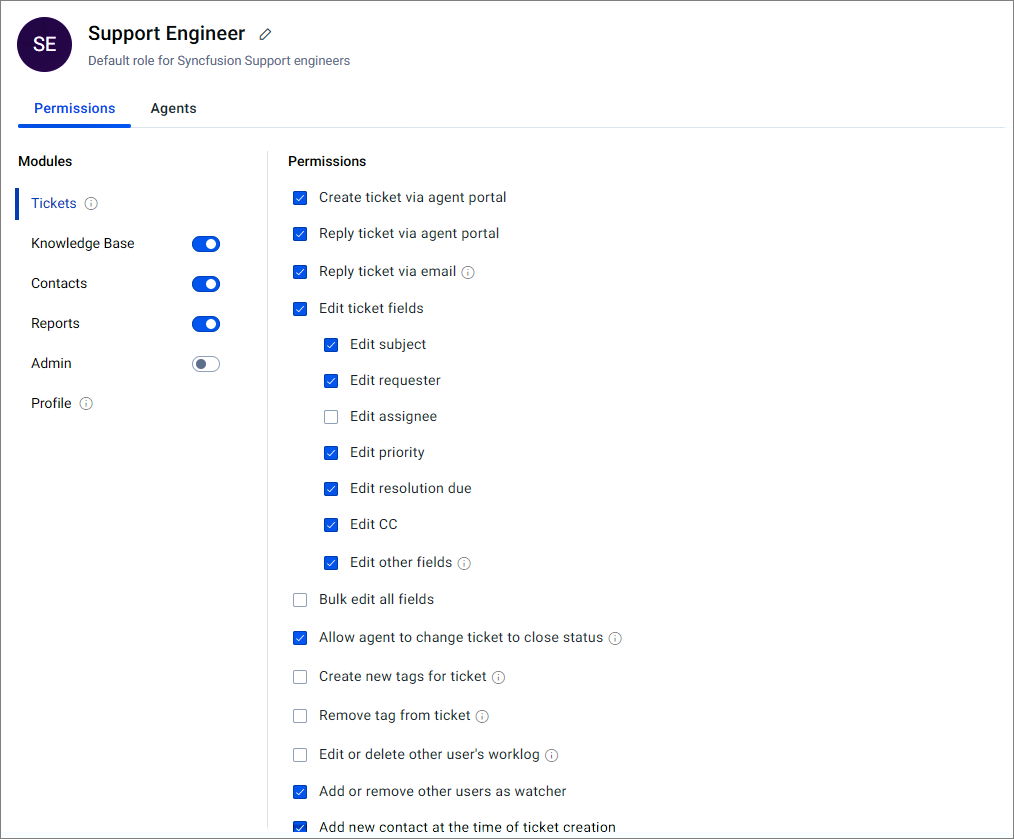This image captures a settings or permissions page of a website or application, likely intended for managing user roles and access. The photo is square in shape with a thin black border surrounding it. At the top, there is a white background coupled with a horizontal gray line about 10% from the top, serving as a header.

In the top left corner, a dark blue circle with white letters "SE" denotes the user role icon. To the right of this icon, in black text, is the title "Support Engineer" followed by an "Edit" button. Below this, there's a description stating "Default role for Syncfusion support engineers."

Two main tabs are present below this section: "Permissions" and "Agents," with "Permissions" highlighted in blue and underscored by a blue line. Beneath this header, the screen is divided into sections. One section labeled "Modules" includes several options. The "Tickets" module is currently selected, indicated by a blue highlight and adjacent vertical blue bar.

The settings within the "Modules" section feature toggle switches for different categories: "Knowledge Base," "Contacts," "Reports," "Admin," and "Profile". The toggles vary in their states; the first three are turned on while the second one is off.

To the right is a detailed listing of specific permissions associated with the role. This section contains various checkboxes, some filled in blue with a white checkmark and others remaining empty. Examples of these permissions include "Create ticket via agent portal" and "Reply to ticket via agent portal." This detailed breakdown likely represents the customizable settings for the role of a support engineer.